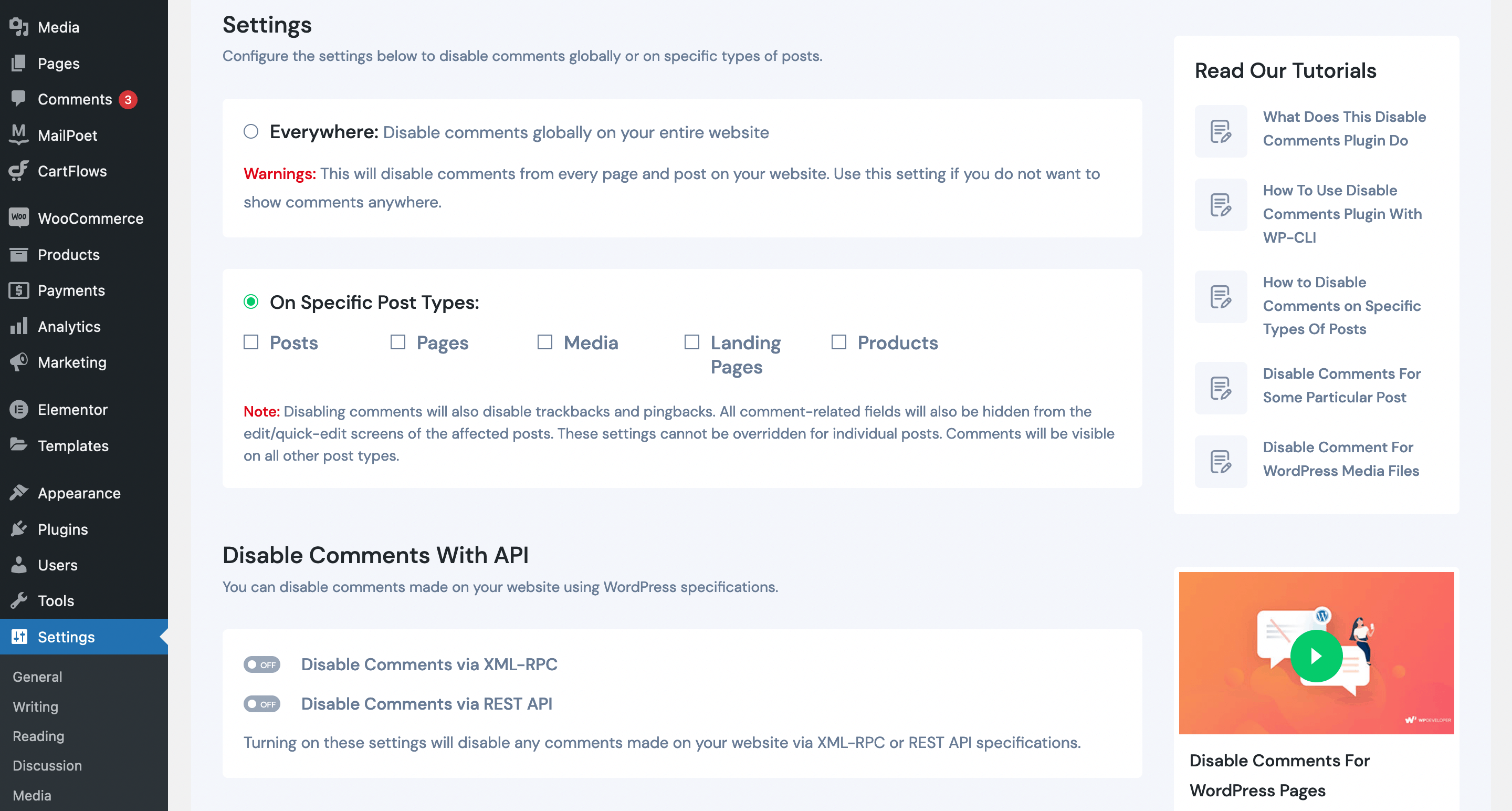Screenshot Description: WordPress Settings Panel for Disabling Comments

This screenshot captures a WordPress settings panel designed for disabling comments on various types of posts. The interface is structured with a gray vertical panel on the left side, featuring a list of options including Media, Pages, Comments, among others. Each of these options is accompanied by an icon, though they are not described in detail.

The "Comments" section is particularly notable, displaying a red notification badge with the number three, indicating that there are three comments awaiting moderation.

Further down the left panel, a host of additional options appear, such as Mail, Post, CartFlows, WooCommerce, Products, Payments, Analytics, Marketing, Elementor, Templates, Appearance, Plugins, Users, Tools, and Settings. The Settings option is highlighted with a blue background, indicating it is currently selected.

Within the Settings panel, several sub-options are listed, including General, Writing, Reading, Discussion, and Media. The main focus of this screenshot is on the configuration settings for disabling comments. The user is presented with options to disable comments globally or for specific post types such as Posts, Pages, Media, Landing Pages, and Products. These settings appear to be customizable, with checkboxes to enable or disable each option. The "Disable Comments with API" options are both turned off.

On the right side of the screenshot, there is a vertical sidebar labeled "Read Our Tutorials," featuring five articles to assist users. Below this, there is a thumbnail for a video tutorial titled "Disable Comments for WordPress Pages," showcasing an orange background and an illustration of a woman sitting on a speech bubble.

Overall, this screenshot provides a detailed view of the settings area within WordPress, focusing specifically on the configuration options available for managing and disabling comments, complemented by tutorial articles and a video. The browser interface is not visible in this screenshot, keeping the focus solely on the WordPress settings panel.